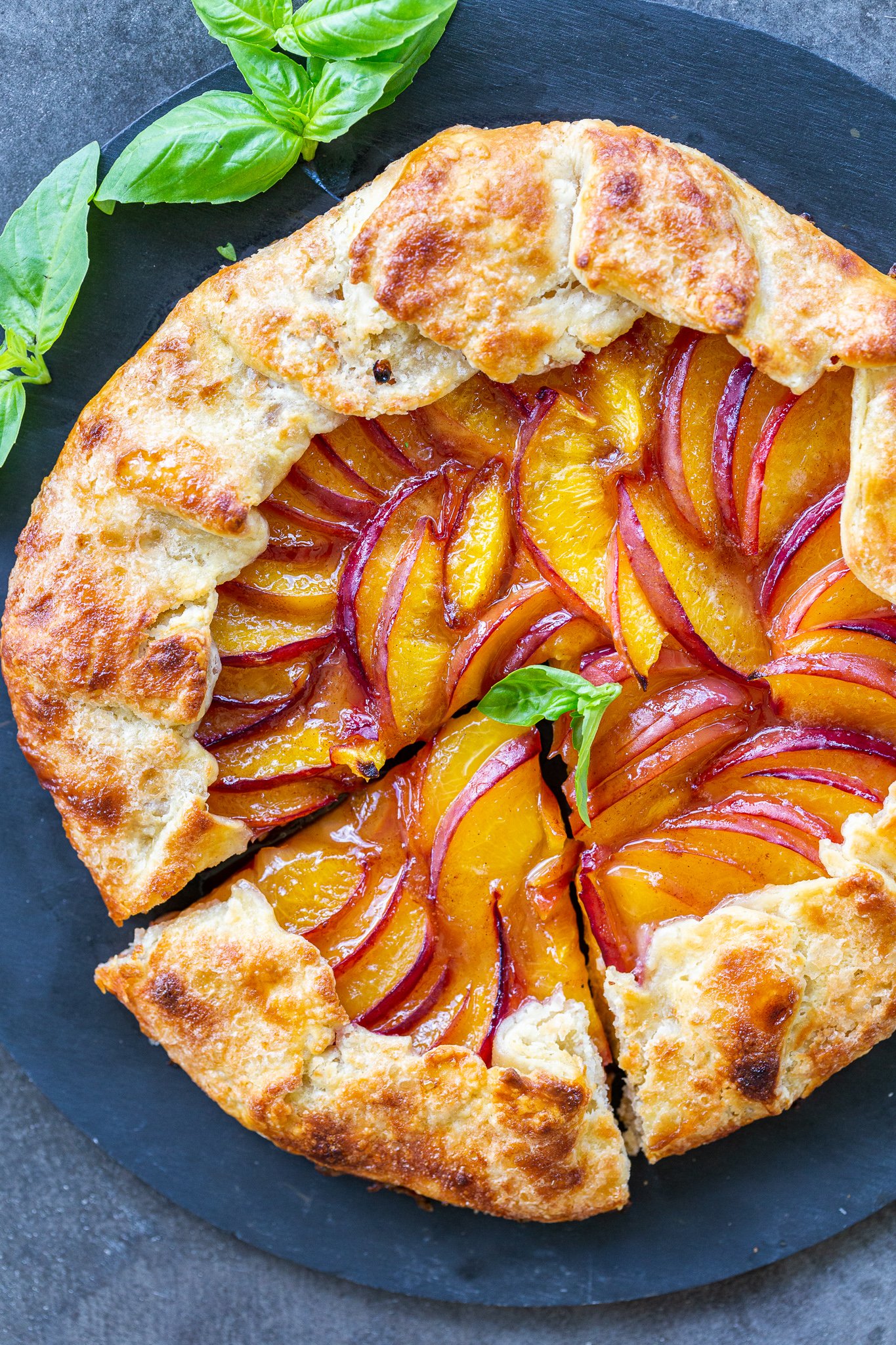This portrait-oriented photograph features a tantalizing dessert, centrally placed on a table with a charcoal gray hue. The focal point is a dark charcoal or black plate, hosting a beautifully crafted galette. The galette's golden-brown puff pastry crust, which appears lightly toasted in an oven, encircles an array of thinly sliced, glazed peaches. The peaches, arrayed in a circular pattern, transition from red on the exterior slices to yellow towards the center, evoking a shimmering, mouth-watering effect. A slice of the galette is slightly pulled away, revealing more of the delectable interior. A sprig of green mint garnish adorns the center of the dessert, while two additional mint sprigs rest in the upper right corner of the plate. This captivating presentation sits on a black plate, adding to the visual allure of the dish.